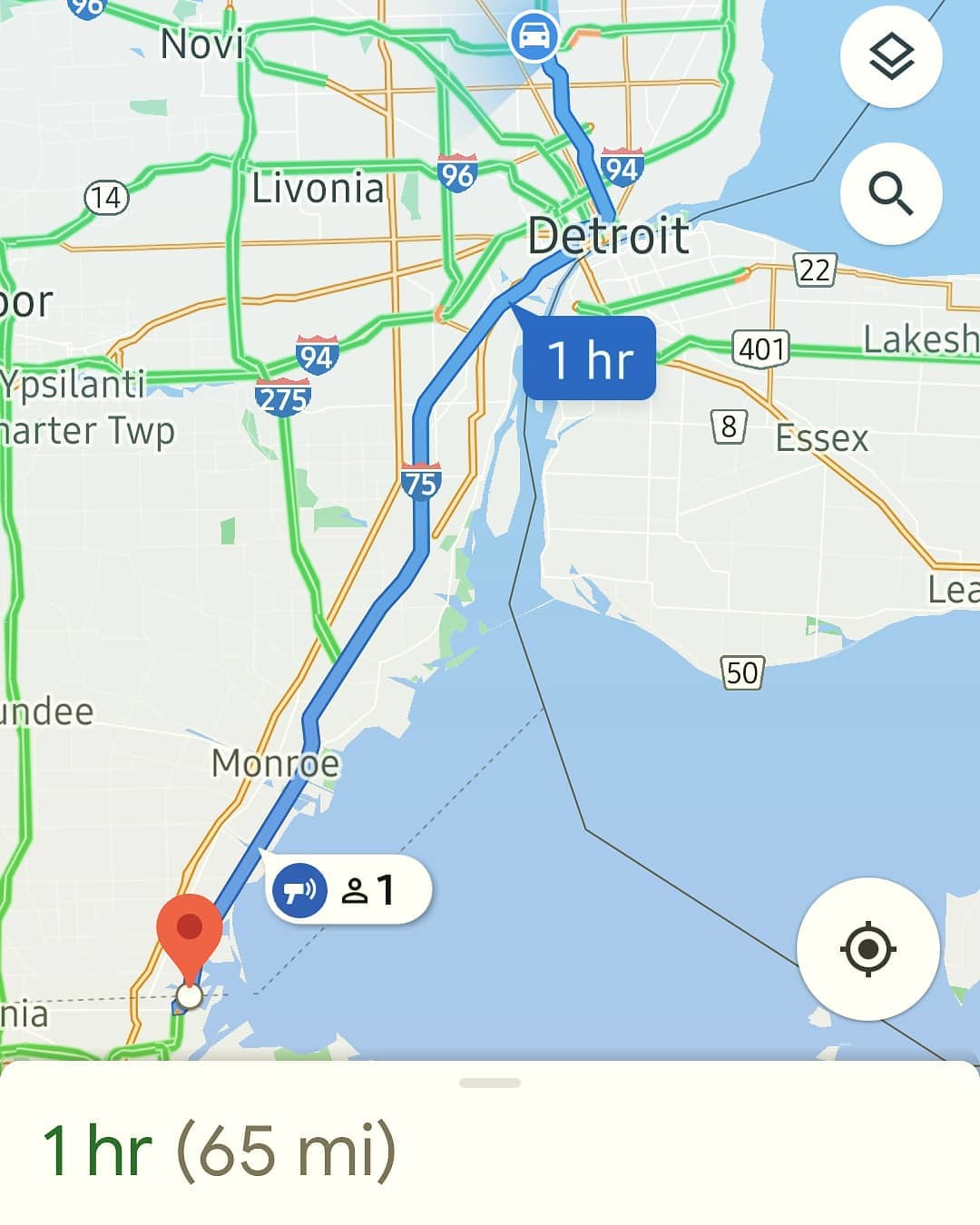This image is a detailed close-up screenshot of a Google Map focusing on Detroit. The central feature is a blue route line that starts from a red pin at the bottom left and travels upward to the top. This route is marked with a bubble that indicates a travel time of "1HR". The route intersects major highways such as I-75, which is highlighted among other roads shown in green and orange, including highway signs for 96, 94, and 275. The land is depicted in white, and the water, including lakes around Detroit, is shown in blue with black lines crossing through it. Notable street names on the map are Essex, Lakeshore, Lenovo, Novi, and Monroe. In the bottom right corner, there's a circle with a bullseye symbol, while the upper right corner features a white circle containing a black square and another white circle with an hourglass beneath it. At the map's bottom left, travel details are reiterated: "1HR (65 miles)." The map also includes a small blue circle with a white car representing Detroit, from where the mapped route begins.